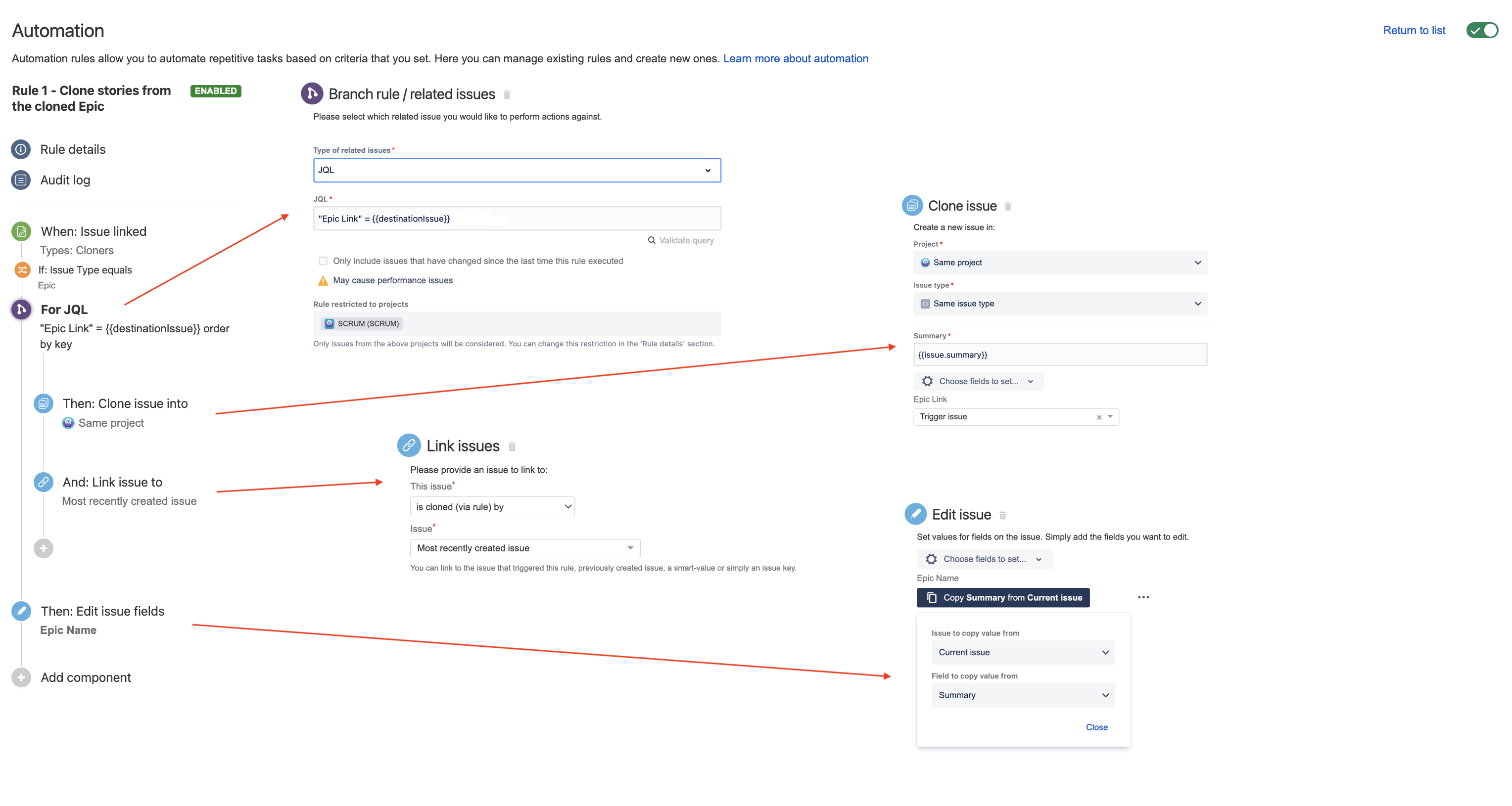This image, taken from a web page focused on automation, features several red arrows highlighting key sections and labels. At the top, the heading "Automation" is prominently displayed. Below this, a subheading explains, "Automation rules allow you to automate repetitive tasks based on criteria that you set. Here you can manage existing rules and create new ones," along with a prompt to "Learn more about automation."

In the main section of the page, Rule One is described as "Clone stories from the cloned epic" and is marked as enabled, indicated by a clickable blue button labeled "Enabled." Subsequent details of the rule are provided under sections labeled "Rule details" and "Audit log."

Various red arrows guide the viewer's attention: one arrow points from an area labeled "For JQL" to the JQL input section, another arrow spans from the "Same project" label to a summary input area, a third arrow connects "Add link to" to the "Link issues" section, and the last arrow directs from "Then edit issue fields" towards a box located at the lower right corner of the page.